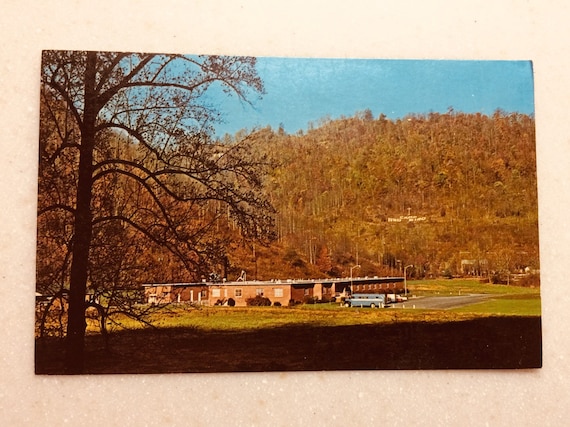This is a detailed photograph likely from the 1960s, showcasing a single-story, flat-roofed brick building that could be a school or government facility. The building is situated in a flat, green field, with a large tree in the foreground. The tree has few leaves, suggesting it is fall. A blue bus is parked directly in front of the building, drawing attention to the mid-ground. The backdrop features a rapidly rising hill covered with a mix of brown, golden-brown, and some green trees, fitting with the autumnal setting. Above this scene is a clear, blue sky. The photograph itself, displayed on a light brown piece of paper, exhibits shades of orange and brown, resonating with the fall season. The shadow spreading over the grass in the foreground suggests the photo was taken in the early evening. All elements combined paint a nostalgic and serene image of rural autumn.